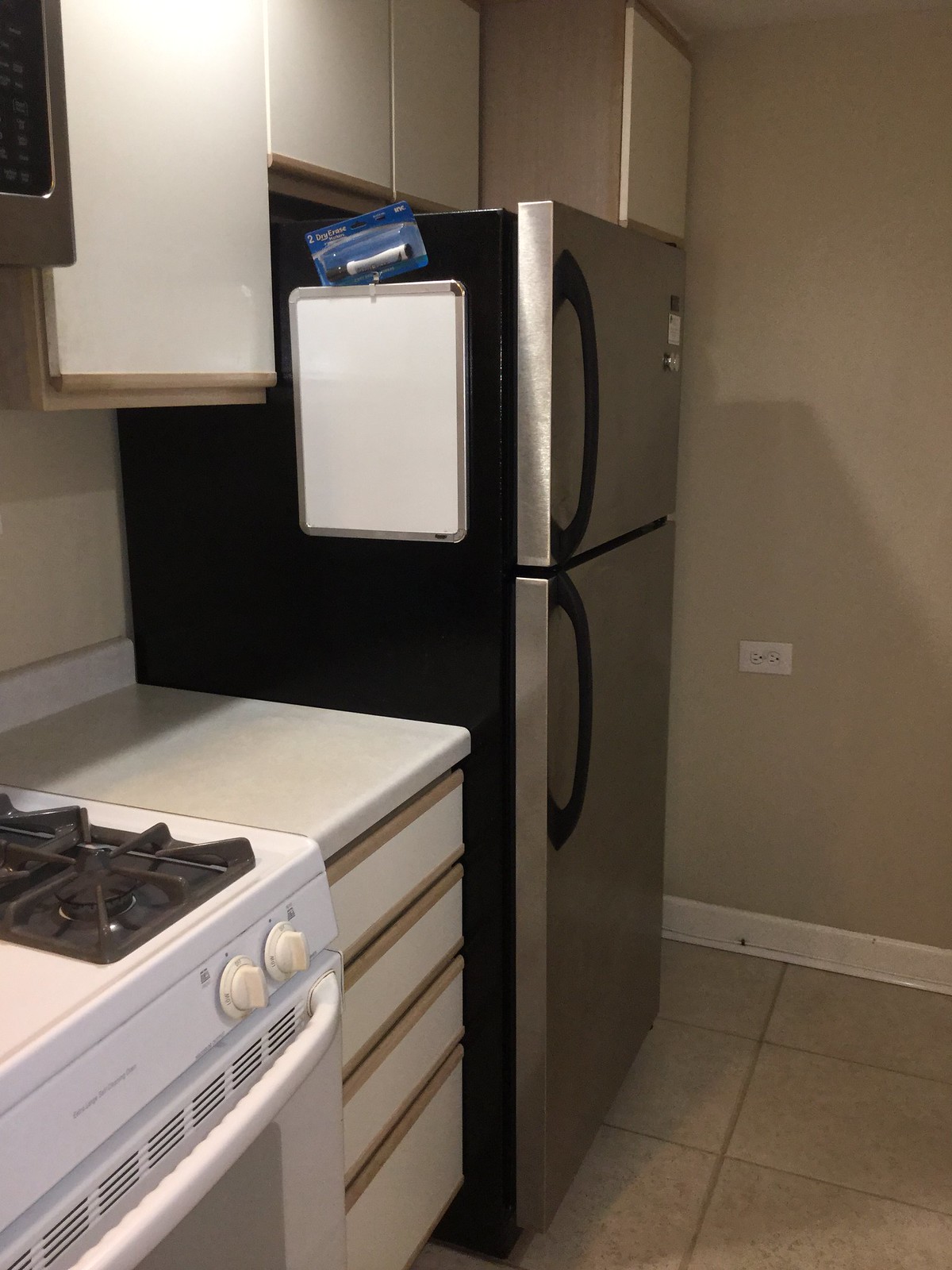This detailed photograph captures a section of a cozy kitchen. The main focus is a refrigerator with a stainless steel door and sleek black handles, positioned centrally for a side view. The side of the refrigerator features a white dry-erase board secured with a magnet, along with a marker stored above it. The surrounding beige walls include a rectangular power outlet. Adjacent to the refrigerator is a white gas stove with prominent dark burners and two white knobs. Above the stove, a microwave is partially visible, attached to the wall's cabinets. The cabinets, combining beige wood and white laminate fronts, complement the kitchen's aesthetic. Below the microwave is a countertop housing black burners. Above and to the side of the refrigerator are additional cabinets, contributing to the kitchen's storage. The floor consists of large, white tile squares. Overall, the kitchen exudes a functional and organized charm, punctuated by thoughtful details.